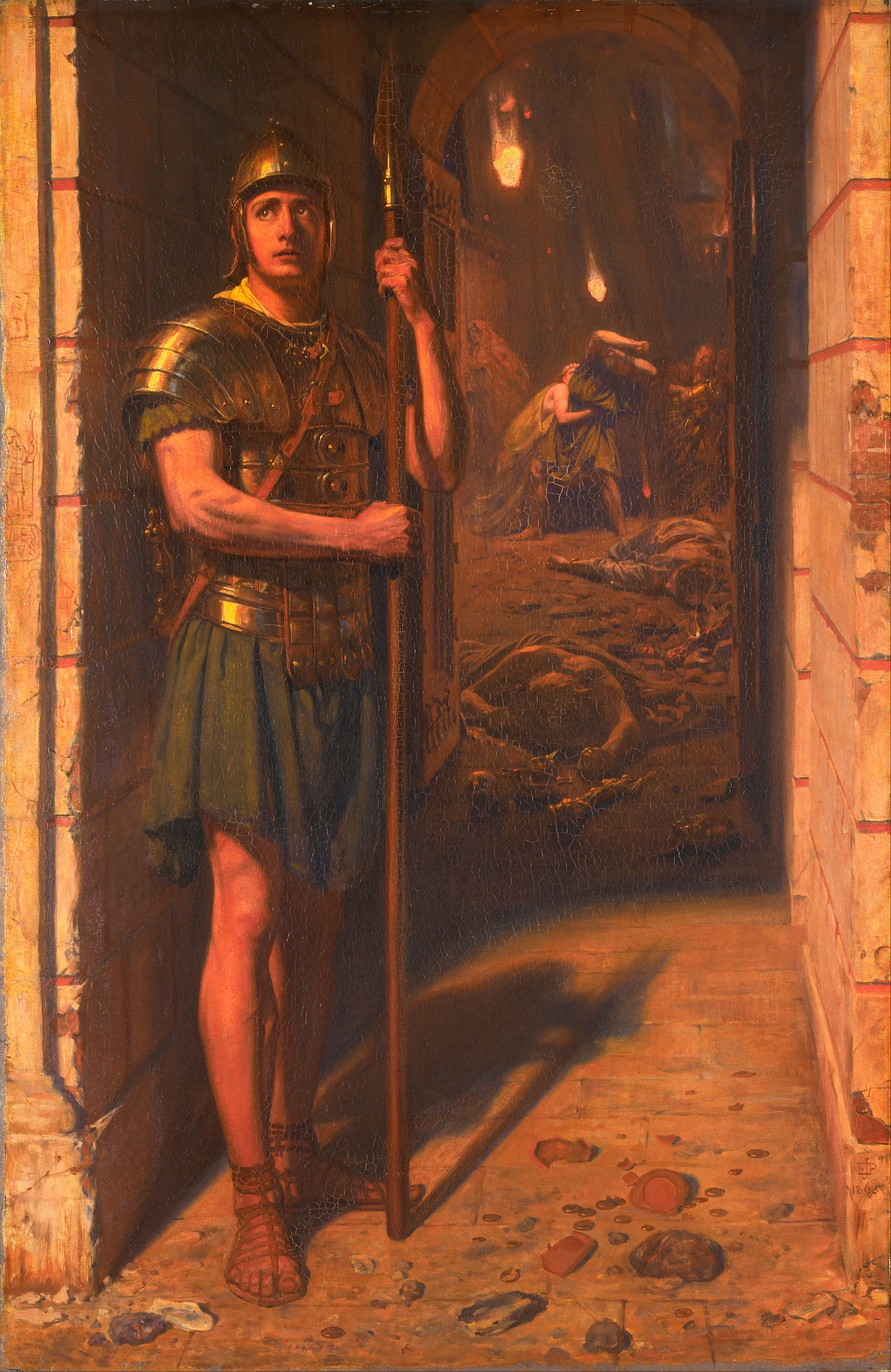The painting, vertically oriented and rich with historical connotations, prominently features a Roman guard standing tall in an archway on the left side. The guard is clad in a metallic breastplate, helmet, and leather sandals, with a dark grey or dark blue skirt. He holds a spear with his left hand higher than his right, gazing sternly towards the right. The sun casts shadows indicating it's shining from outside the archway into the dim interior. This warm-toned oil painting, with muted browns, golds, and yellows, plunges into a chaotic and violent scene within the interior space. Bodies are strewn across the floor, some appearing lifeless, while others depict a woman clinging to a man amidst the turmoil. Several people are seen cowering and shielding their faces as flaming rocks and debris cascade down upon them, adding to the sense of disaster and commotion. This rich tableau suggests an event of gladiatorial combat, a prison riot, or some other Roman era chaos, blending scenes of valor and violence into a striking historical narrative.